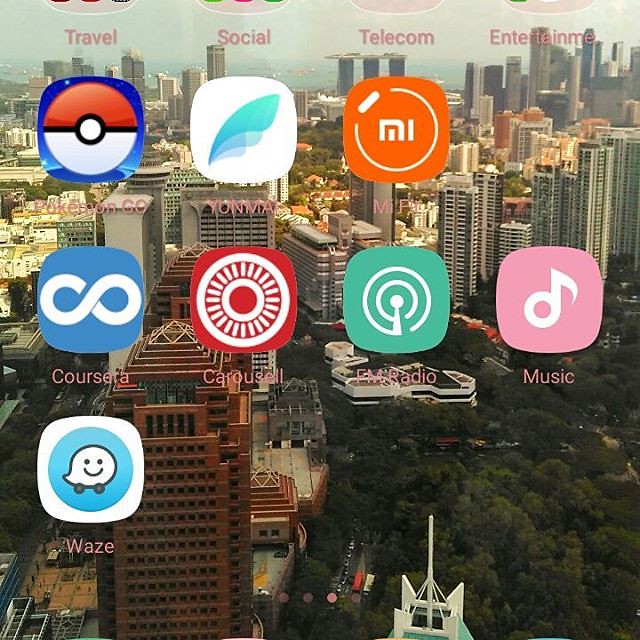The image depicts a vibrant cityscape with towering buildings and a sprawling park situated in the lower right corner. Superimposed on this urban scene are various app icons, creating a digital overlay on the photograph. The app icons visible include Pokemon Go, Yanma (or possibly Yanmai), Me, F, Coursera, Carousel, FM Radio, Music, Waze, and Me Fit. Above, some additional app icons appear grayed out, blending subtly into the backdrop.

The icons are typical of those found on mobile devices, representing common applications. Some names and icons are partially obscured due to the busy background, making them difficult to discern clearly. The text beneath the icons is in a light pink hue, adding to the challenge of readability against the white and light-colored buildings.

Given the large, square format of the display, it is likely that the image was captured or displayed on a tablet device, such as an iPad, rather than a smartphone.